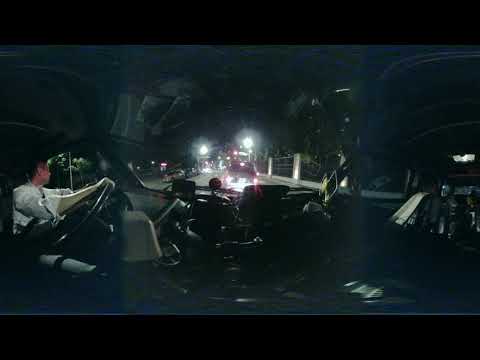In a 360-degree view taken from inside a dark vehicle, the center frame shows a dashboard perspective looking out onto a dimly lit road with several blinding street lights ahead. The left and right views join to provide a complete panoramic image. On the left, a man with dark hair, dressed in a white shirt with a slightly greenish undershirt and white pants, is seated in the driver's seat, his hands on the steering wheel, looking out the window to his left. Visible in the background are some green foliage illuminated against the night sky. To the right and behind the car, multiple parked vehicles can be seen, including a light gray and a black coupe. There are additional details in the center view, such as a tow truck suggesting that the vehicle is possibly on the back of this truck, and the road is lined with a fence and parked cars on either side. The interior is prominently dark, populated with various cameras and tools, indicative of a front and rear dash camera setup capturing the scene.